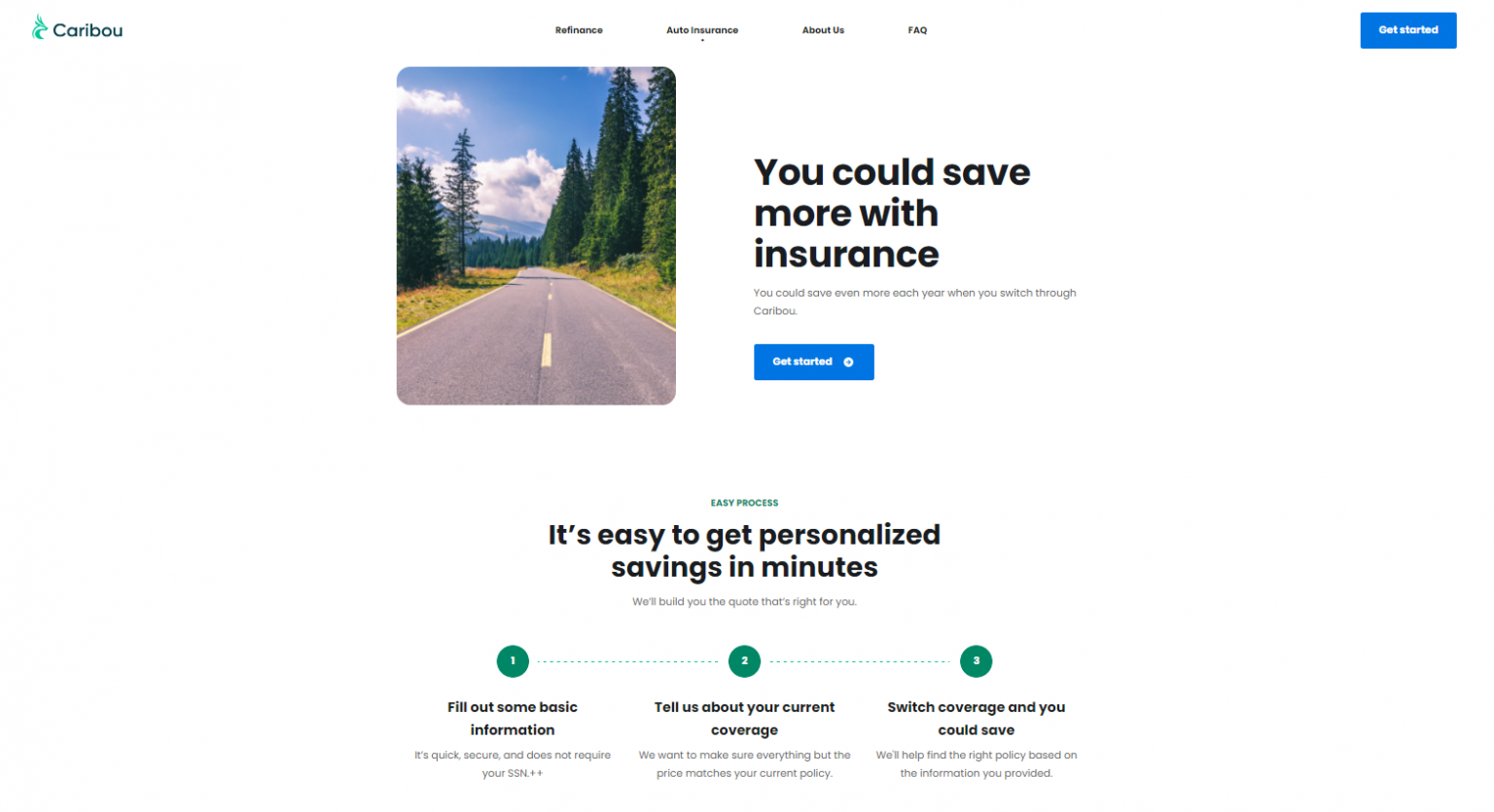The image is from a website promoting insurance services. In the upper left-hand corner, the word "Caribou" is prominently displayed in bluish-green text. Adjacent to this logo, there are several categories listed in sequence: "Refinance," "Auto Assurance," "About Us," and "FAQ." On the far right side, there is a blue rectangular button with white text that says "Get Started."

Beneath the "Refinance" category, there is a scenic photograph featuring a paved road stretching through the countryside. The perspective places the viewer in the middle of the road, with lush green grass flanking either side and a backdrop of tall fir trees. The sky overhead is a vibrant blue dotted with fluffy white clouds.

To the right of this picturesque scene, bold text proclaims, "You could save more with insurance," followed by another blue "Get Started" button. Below this, black text reassures visitors that "it's easy to get personalized savings in minutes."

Further down, three steps guide prospective customers through the process, marked by numbered points in small green circles: 

1. **Fill out some basic information.**
2. **Tell us about your current coverage.**
3. **Switch coverage and you could save.**

The layout and design elements aim to create a user-friendly experience, encouraging visitors to take action and explore potential savings on their insurance.